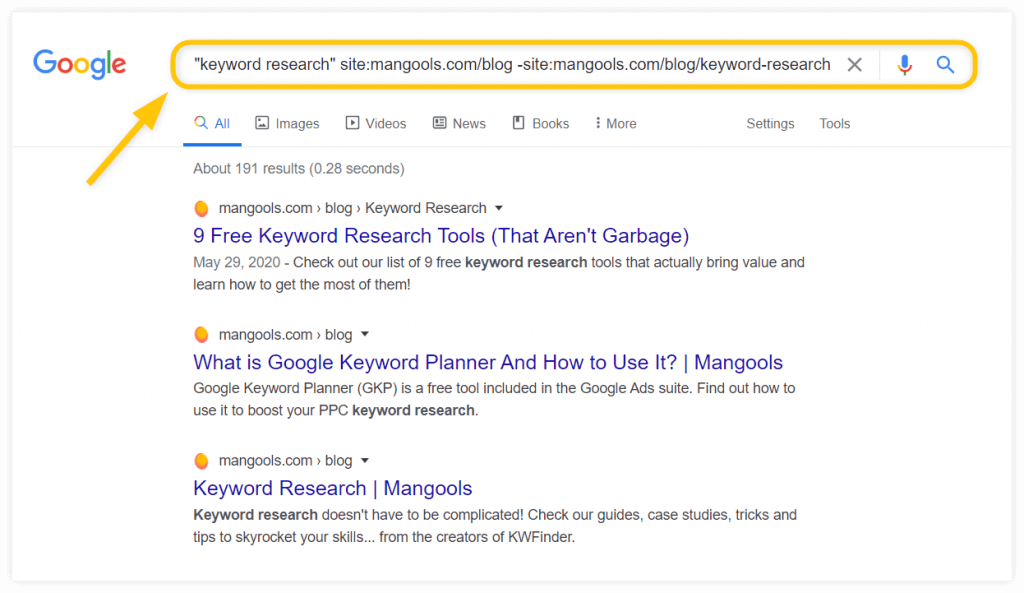This photo captures a Google search results page in detail. At the top left, the word "Google" and the Google logo are prominently displayed next to a search bar circled in yellow with a yellow arrow pointing to it. The search query entered is “keyword search site:mangoles.com/blog -site:mangoles.com/blog/keyword-research”. Beside the search bar, the 'X' icon for clearing the query, the microphone icon for voice input, and the magnifying glass icon for initiating the search are all visible.

Directly below the search bar is a navigation menu including options for "All," "Images," "Videos," "News," and "Books," followed by a "More" dropdown. To the right, "Settings" and "Tools" options are available. The search has yielded approximately 191 results. The highlighted first result is an article titled "Nine Free Keyword Research Tools That Aren’t Garbage."